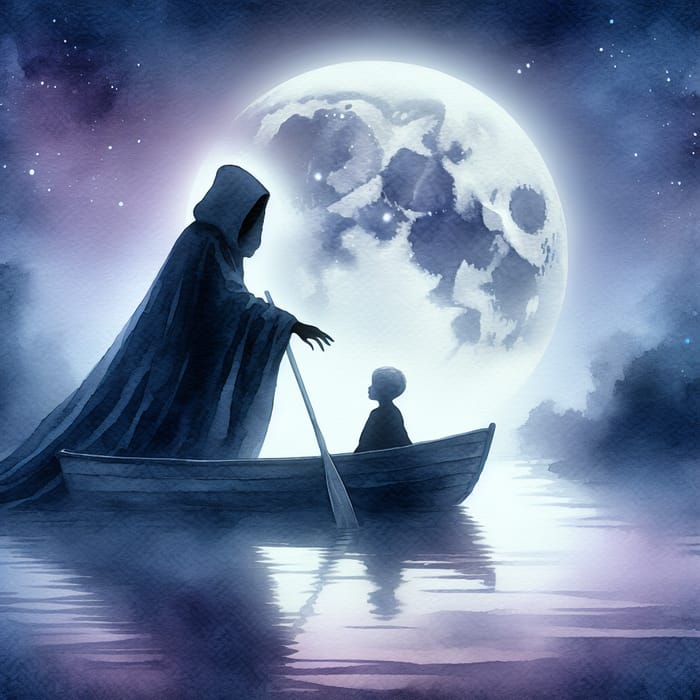In this detailed watercolor illustration, we observe a surreal nighttime scene set on a still pond, captured in a square format. The focal point is a small wooden rowboat containing a young boy seated and looking upwards, seemingly in a state of vulnerable anticipation. Opposite him stands a tall, enigmatic figure cloaked entirely in dark robes, reminiscent of a Grim Reaper but open to various interpretations such as a ghostly or even divine presence. This figure, shrouded with a hood, extends one hand toward the boy while gripping an oar with the other. Dominating the background is a large, luminous moon that illuminates the scene, surrounded by an ethereal mix of purple and gray clouds. The star-studded sky adds to the mystical atmosphere, and the bright moonlight casts shimmering reflections on the water's surface, enhancing the painting’s dreamy, almost otherworldly, ambiance. The overall composition fuses elements of serenity and suspense, drawing the viewer into its enigmatic narrative.